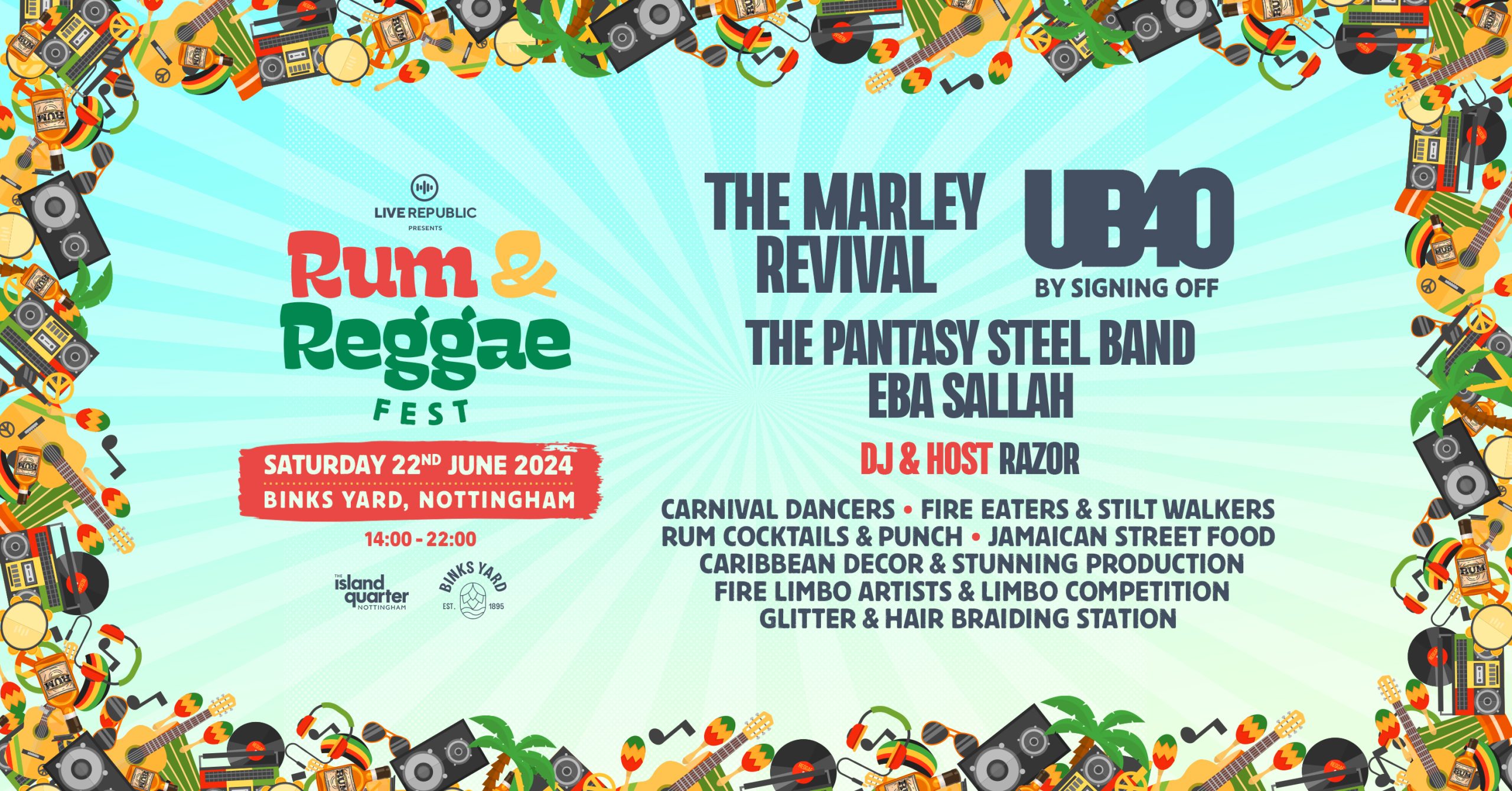The advertisement poster for the Rum and Reggae Fest features a vibrant, starburst background shaded in blue and light blue hues. The border is adorned with reggae-themed instruments and iconography, such as palm trees, speakers, guitars, records, turntables, maracas, and musical notes, all incorporating the colors of the Jamaican flag. Central to the poster is bold text announcing "Rum & Reggae Fest" with "Rum" in red, the ampersand in yellow, and "Reggae Fest" in green. The festival, hosted by Live Republic, is scheduled for Saturday, June 22, 2024, at Bink’s Yard, Nottingham, from 2 p.m. to 10 p.m. The headliners include The Marley Revival and UB40 by Signing Off, with additional performances by The Pantasy Steel Band, Iba Salah, and DJ and Host Razor. The event promises a lively atmosphere with carnival dancers, fire eaters, stilt walkers, rum cocktails, punch, Jamaican street food, Caribbean decor, fire limbo artists, a limbo competition, and a glitter and hair branding station. The poster also features logos for Island Quarter and Bink’s Yard.